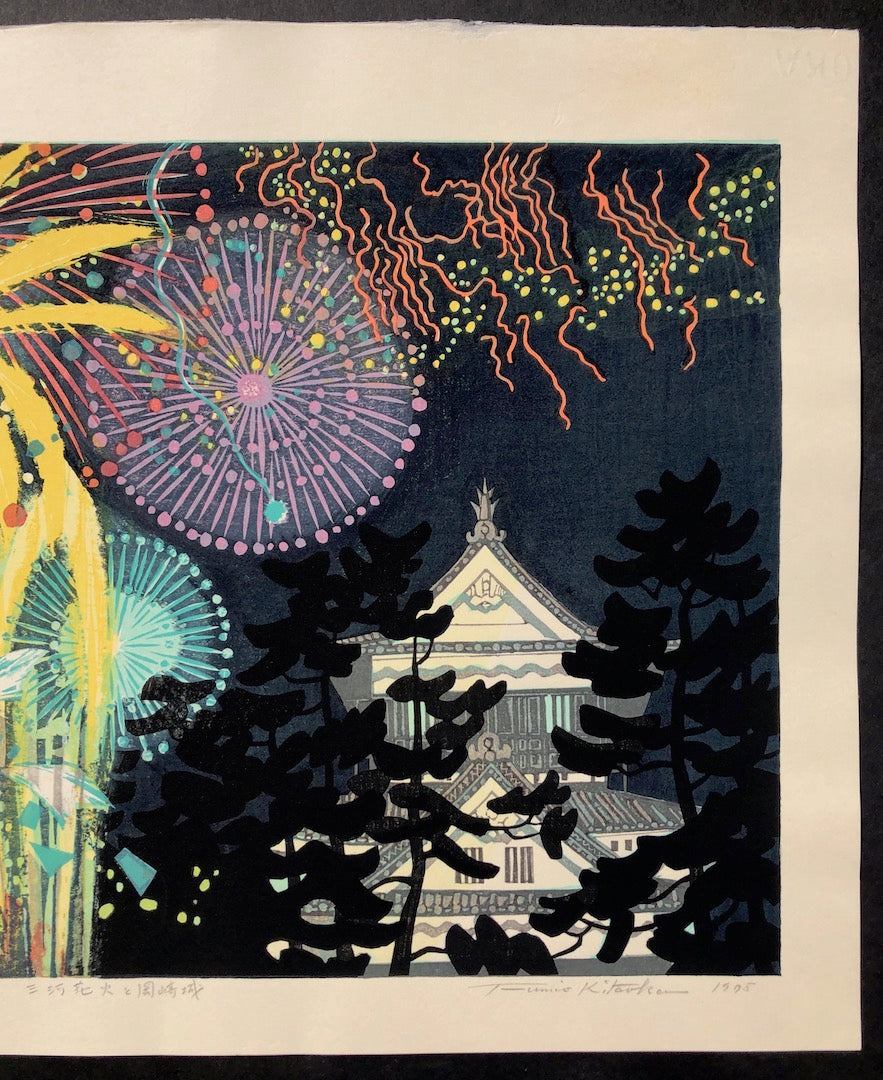This is an artistic photograph of a framed print depicting a stylized night scene. The image, truncated on the left, features a white and slate-blue house with a pagoda-like architecture shrouded among trees. Above the house, a dark midnight-blue sky is illuminated by an array of colorful fireworks. These fireworks create circular bursts primarily in purple and teal blue, with splashes of yellow and dots of red and orange, along with yellow dots scattered across the sky. Falling ribbons of orange add to the vibrant display. The scene is framed with a light cream border adorned with indistinct handwriting along the bottom edge, and this is surrounded by a thicker black border. The artwork, likely a print or a poster, has an abstract feel, capturing the festive charm of fireworks over an oriental-style house.